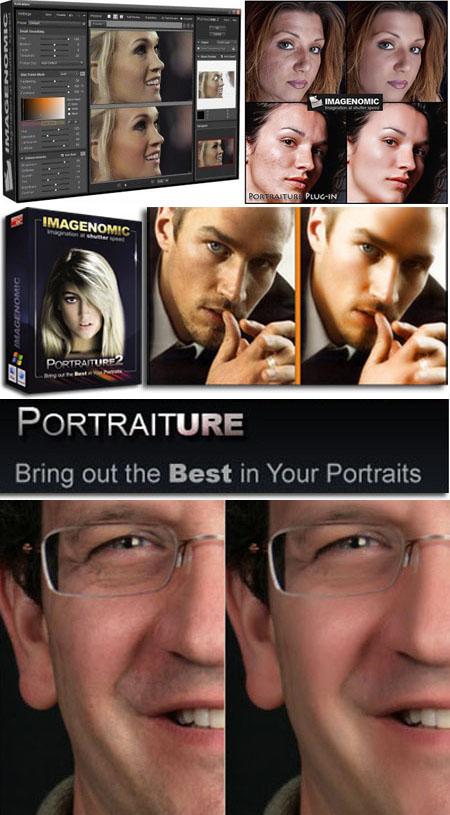This image appears to be an advertisement for a professional image editing software called "Portraiture" by ImageNomic. Dominating the layout are side-by-side comparison photographs showcasing the software's prowess in enhancing portraits. Featured prominently is a man whose "before" image on the left is markedly improved in the "after" image on the right. Similarly, another set of photos of a woman with blonde hair highlights the transformative effects of the software, emphasizing clearer, retouched results.

In the upper right section of the advertisement, four additional photographs are stacked vertically, further illustrating the software's capability with two "before" shots on the left and their significantly improved "after" counterparts on the right. 

The text prominently features the tagline "Bring out the best in your portraits" in white letters, reinforcing the software’s main selling point. The ImageNomic logo appears boldly in yellow, further establishing the brand. The color scheme of the ad primarily utilizes black, white, skin tones, and hints of yellow and pink. Additionally, the bottom of the advertisement displays a box showing product details, although the fine print isn't legible, which likely includes additional information and testimonials.

Overall, the advertisement successfully conveys the message that Portraiture by ImageNomic is a robust tool for enhancing portrait images, making them clearer and more refined.